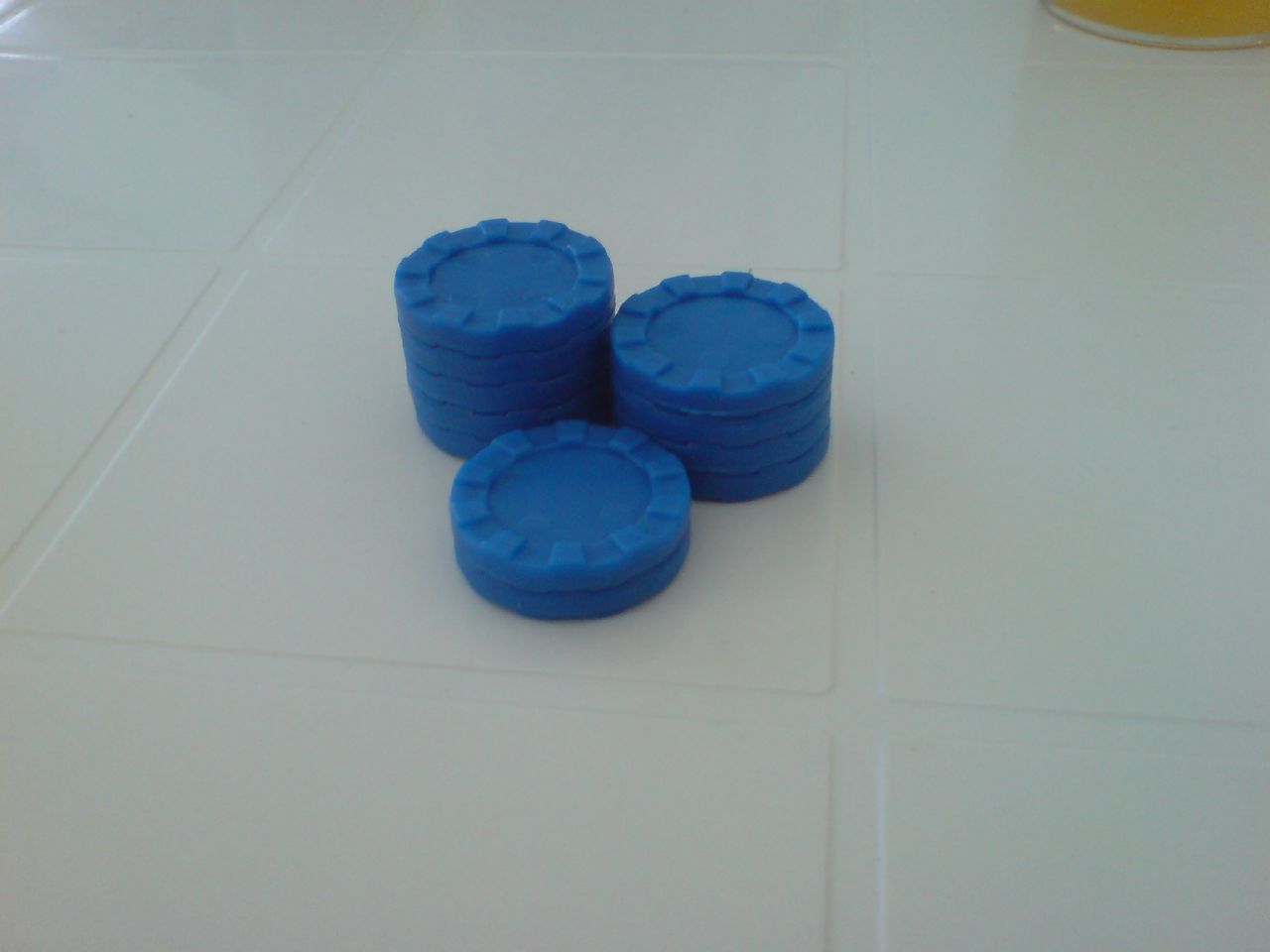The image features a white, glossy, tiled countertop with distinct square tiles and visible white grout lines. Reflective light can be seen on the surface, particularly in the upper section. Centrally placed on the countertop are three neat stacks of blue casino chips, totaling eleven in number. The stacking arrangement includes a front stack of two chips, a middle-left stack of five chips, and a middle-right stack of four chips. In the top right corner, partially encroaching into the frame, there is a glass jar or bottle with a yellow body and a white trim at the bottom.